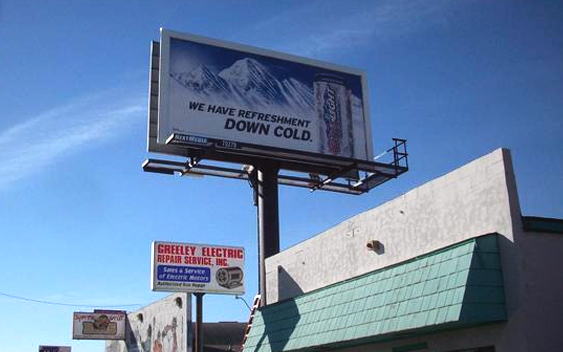This image captures a vibrant streetscape of a small town, focusing on rooftops and storefronts along the main street. Central to the composition is a prominent concrete block building with a distinctive green awning, lacking any visible signage. Above this building, a large billboard—mounted on a tall, black metal pole—advertises Coors Light beer with the slogan "We Have Refreshment Down Cold" displayed in bold black text against a backdrop of snowy mountains and a beer can. Adjacent to this advertisement, a smaller white billboard promotes Greeley Electric Repair Service Incorporated, featuring red text and a blue rectangle stating "Sales and Service." Further along the street, another cement building with an indistinct sign is visible, followed by the faint outline of a partially-obscured sign. The scene is set against the backdrop of a clear blue sky with a wisp of cloud stretching from left to upper right, enhancing the small-town charm of the image.